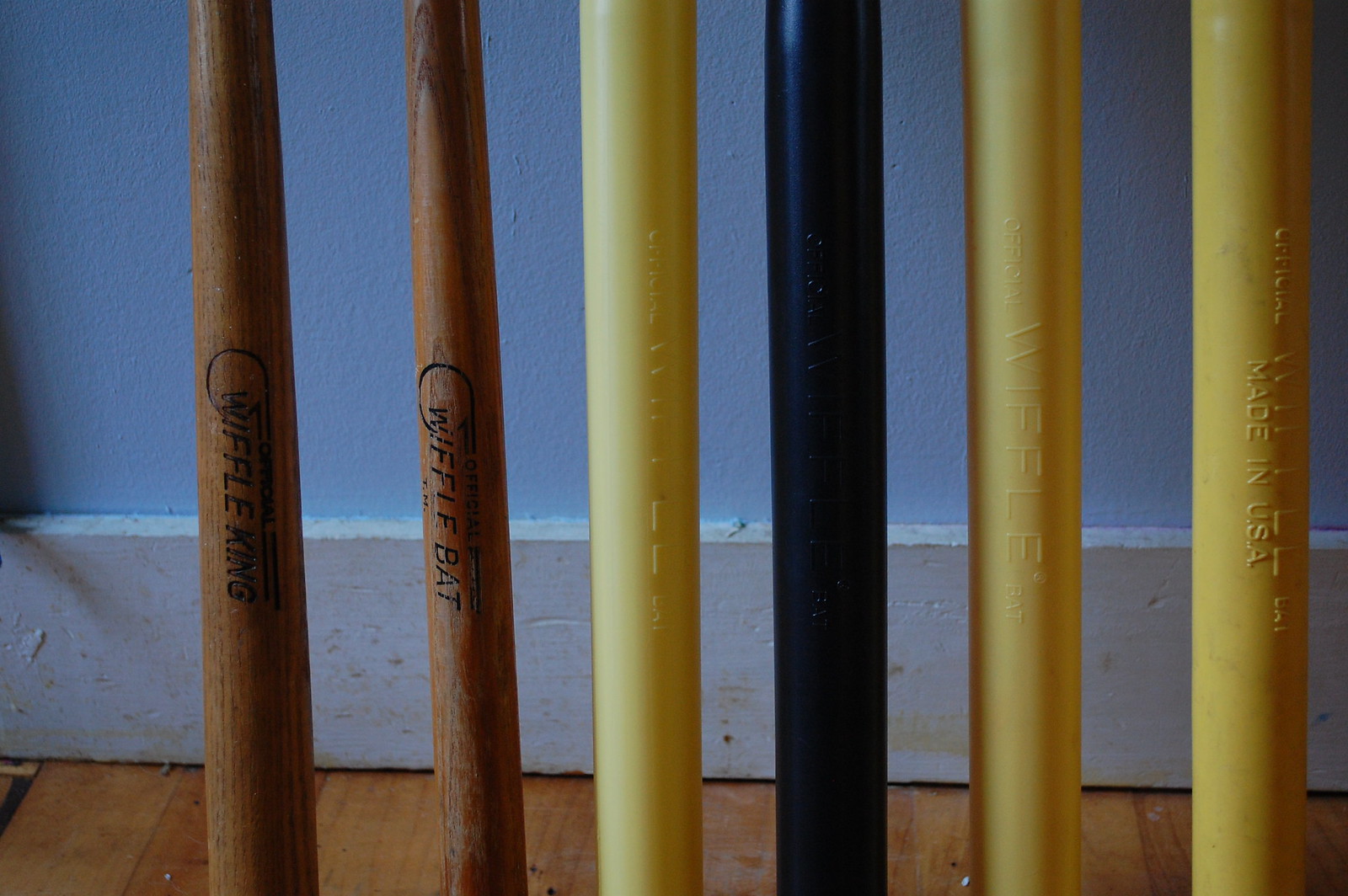This indoor photograph, taken in poor lighting, showcases an intriguing collection of six whiffle ball bats arranged vertically against a pale blue wall with a white, somewhat scuffed baseboard. The floor beneath them is a polished light wood, possibly pine. The two wooden bats on the far left are inscribed with "Wiffle King" and "Wiffle Bat." Meanwhile, the other four bats are plastic, with three being yellow and one black, each marked with "Wiffle Bat" and "Made in USA." The bats are evenly spaced and appear to be standing upright on their own without leaning on anything. The image captures both the uniqueness of the wooden whiffle ball bats and the more common plastic variants, emphasizing the nostalgic and eclectic nature of this collection.